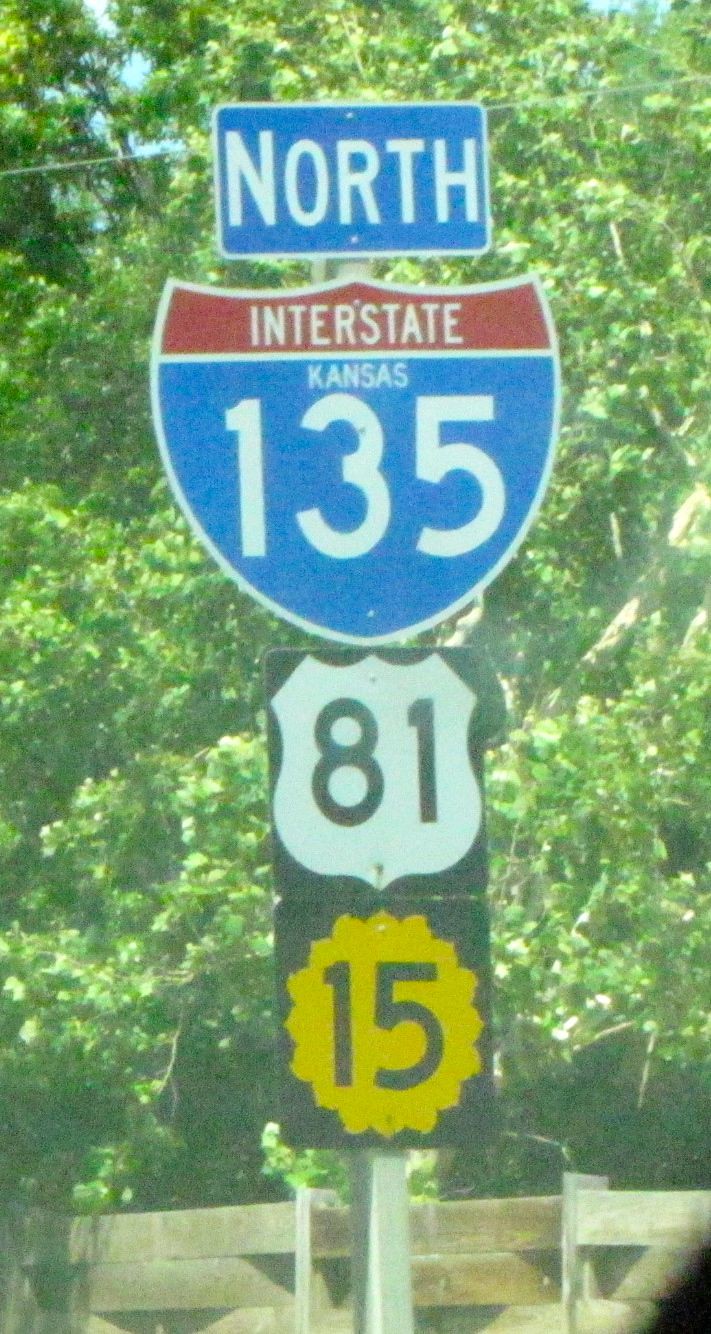The image captures a detailed view of a street sign mounted on a grayish pole. At the top of the sign is a blue rectangular box with "NORTH" written in bold, white capital letters. Directly beneath this is an interstate shield sign, colored red at the top with the word "INTERSTATE" in white. Below that, in the same shield, "KANSAS" is inscribed in white letters, followed by the number "135" in large, prominent white text. Just under this is a smaller, black sign with a white shield outline and the number "81" in black. Beneath this, there is a yellow sun-shaped icon contained within a black square, featuring the number "15" in black. In the background, trees are visible along with a power line crisscrossing the scene. At the bottom of the image, a wooden fence can be seen, providing a rustic element to the setting.